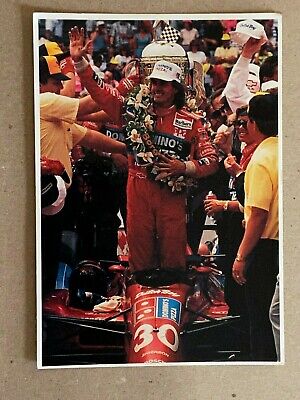The image is a color photograph printed on a light tan, possibly cardboard-like, or a light gray and slightly grainy background with a white border. It captures a triumphant moment of a man standing up in the cockpit of his red race car, which features a prominent white number 30 and a Pizza Hut logo. The car appears low to the ground, reaching just above his knees. The man, clad in a red driving suit with a Domino's logo across the chest and a white cap, is celebrating a victory, likely having just won a significant race such as the Indy 500, judging by his joyful expression and the grand atmosphere. With a floral wreath draped diagonally across his shoulder, he raises his right arm with an open palm forward, holding a bunch of flowers close to his chest with his left hand. The scene around him includes jubilant supporters, with the two closest men in yellow short-sleeved shirts and caps. Behind him, amidst a backdrop filled with flowers, another hand holds up a white cap, while a silver object with a small black-and-white checkered flag can be seen overhead, possibly indicating a trophy. The overall ambiance harks back to the 70s or 80s, adding a nostalgic touch to the image.